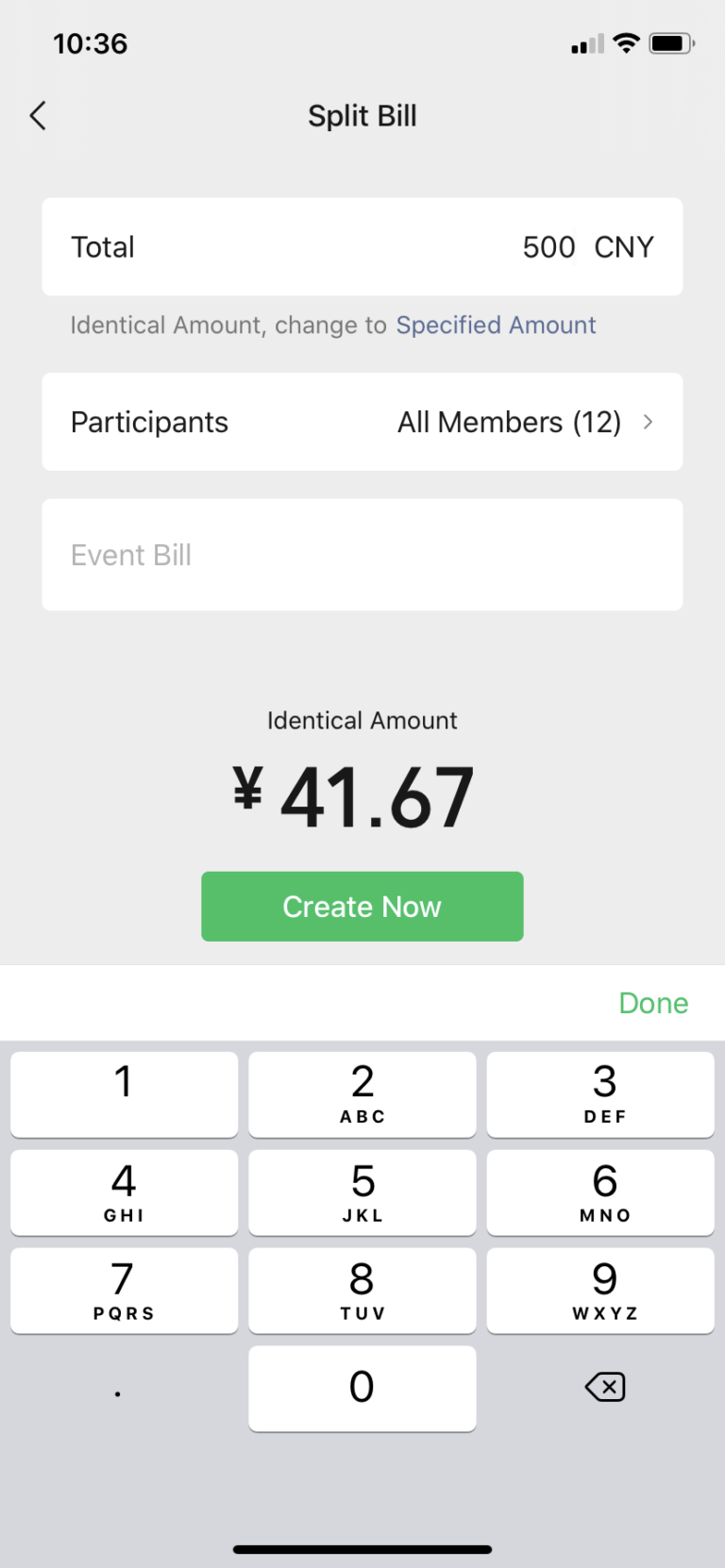Captured at 10:36 AM, this mobile screenshot showcases a split bill interface. At the top right, there are two icons next to a battery indicator. Centered just below, the title "Split Bill" is displayed next to a left arrow. The main section features three distinct white boxes. The first box details the total bill amount as "500 CNY" on the right, with the label "Total" on the left. Below this, instructional text reads "Identical amount change to specified amount." The second box lists "Participants (12)" with a right-pointing arrow. Underneath, labeled "Event Bill."

Lower on the screen, set against a light gray background, the center displays the text "Identical amount" along with a currency symbol and the value "41.67 CNY." A prominent green "Create Now" button appears below this, with a "Done" button situated to the bottom right.

The footer of the screen, also on a gray background, features a numeric keypad. The numbers are arranged with 1-2-3 at the top row, followed by 4-5-6, then 7-8-9, and 0 at the bottom. To the left of the keypad is a left arrow, and beneath the '9' button lies an 'X' icon. A thin black horizontal line bisects the footer section.